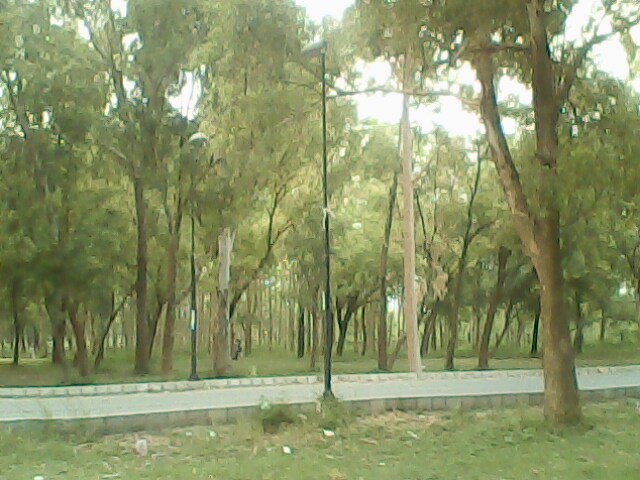The image depicts a somewhat blurry scene, resembling an oil painting, of a forested area with a paved road cutting horizontally across the center. Tall trees dominate the frame, their tops extending beyond the upper edge of the picture, while a bright, white-ish sky peeks through the foliage. The ground in the foreground features flat, grassy areas flanking the road. This road’s curb consists of a series of grayish stones, slightly raised, that would cause a bowling ball to bounce back and forth. Two black light poles, standing about halfway as tall as the trees, are positioned along the road. The predominant colors in the image are green, light and dark brown, gray, black, and white, giving the scene a greenish-brown wash. The overall setting is a forested area outdoors in the middle of the day.